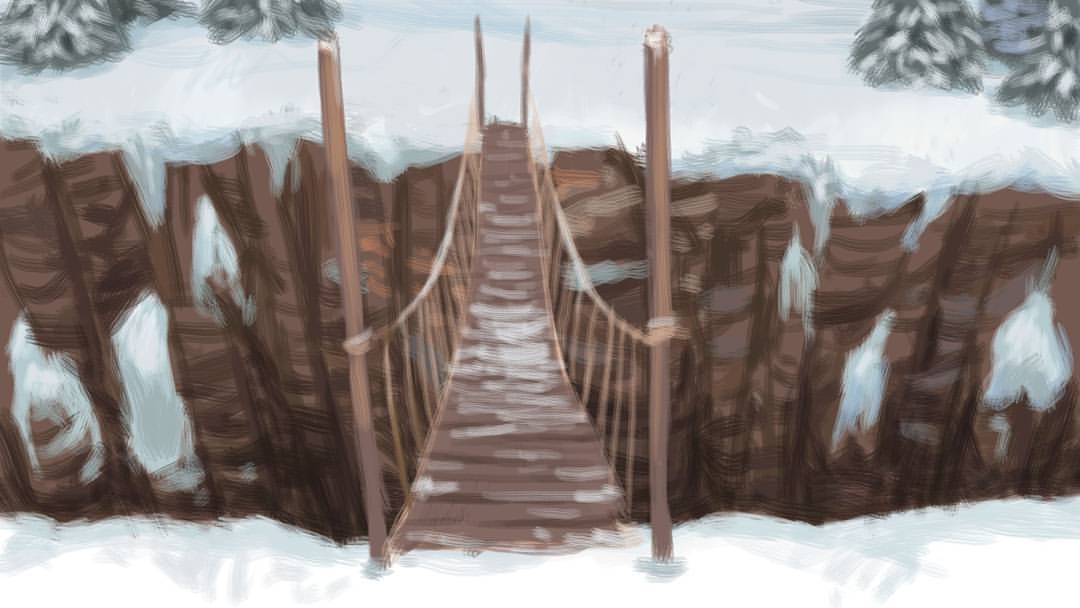The image appears to be, either a detailed painting or a blurred photo of a winter scene. In the foreground, we see a snowy landscape stretching across the bottom of the image. A rickety wooden footbridge extends from this side of the frame, suspended precariously over a deep ravine or crevice. The bridge is supported by ropes tied to sturdy posts on both ends, giving it a fragile and unstable appearance. Snow and ice blanket the bridge, suggesting it might be hazardous to cross. On the far side of the ravine, the snowy ground continues, interspersed with a few pine trees burdened with snow, their presence adding a sense of isolation and cold to the scene. The edges of the cliffs are laden with sheets of ice and snow, reinforcing the cold, wintry atmosphere. The overall composition, with its detailed snowy elements and the precarious bridge, evokes a challenging yet serene wilderness.